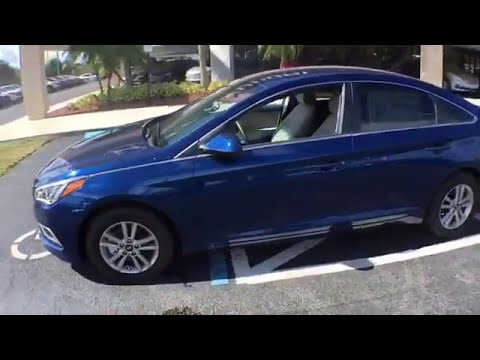This outdoor image captures a compact, royal blue, four-door sedan with a rounded roof and aluminum wheels. The car's gray interior is partially visible through the open driver's side window, while the back passenger window appears tinted. It is parked on pavement marked with white and blue lines, possibly designating a handicap parking space. The setting includes columns of a white building or parking structure with several other cars lined up in rows both underneath and in the background. Tall palm trees and a clear, bright daytime sky are visible, framing the scene and hinting at a possibly warm, sunny location, such as a hotel or shopping strip mall.